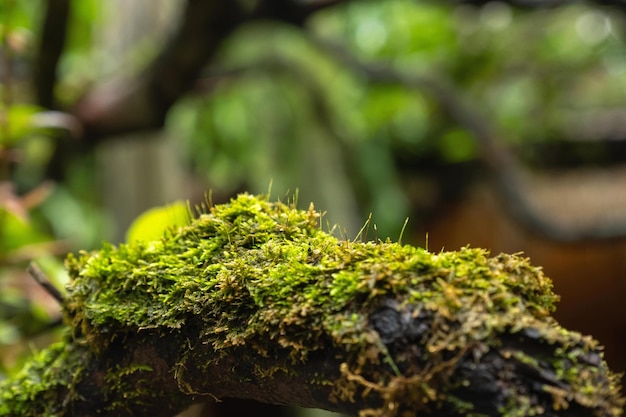This highly detailed, photorealistic close-up captures a moss-covered branch in exquisite clarity. Dominating the foreground, the branch stretches from the bottom left, curving slightly upward to the center before descending to the bottom right. Enveloped in vibrant, bright green moss on its top surface, the branch features evenly dispersed green and yellow sprigs. Along its sides, fringed black and brown leaves add texture, hinting at decayed moss. A smaller, blurry branch juts up to the left, adding depth to the composition. The blurred background offers a glimpse of green leaves scattered across the scene and a black silhouette of another branch that arcs upward and then down to the center-right, exiting the frame. The overall atmosphere is enriched by the soft focus, emphasizing the intricate details and lush color of the moss, contrasting against the subtler hues in the background.